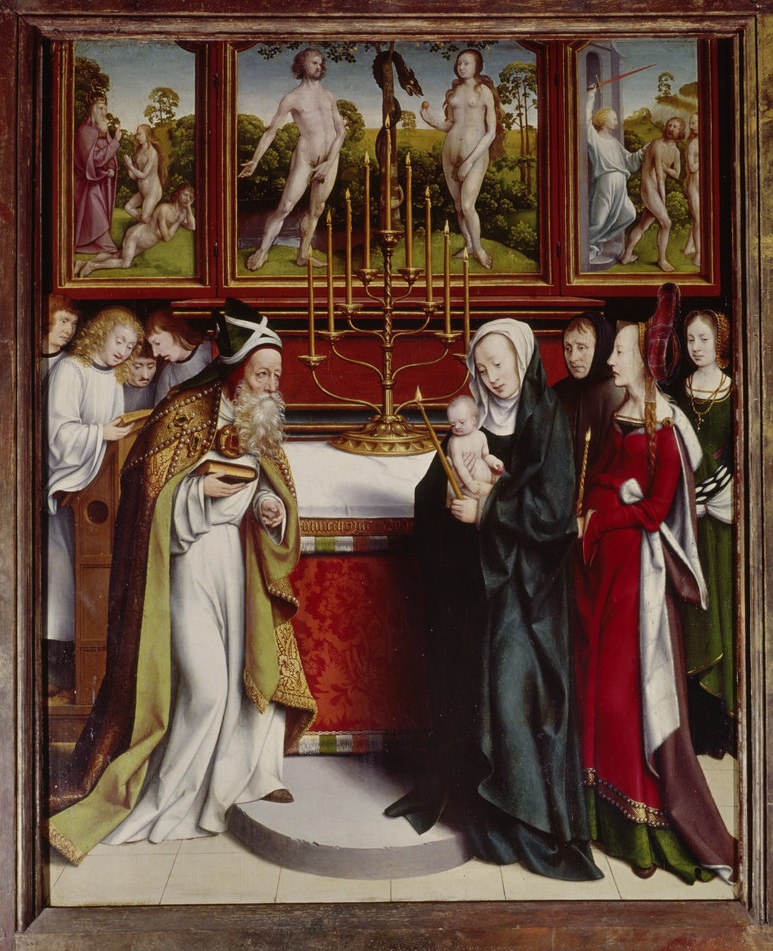This detailed artwork, painted in a Renaissance style, is vertically aligned and resembles the interior of a chapel. The scene is divided into distinct sections with ornate details. At the top, a border resembling a wooden picture frame encloses narrow vertical rectangles on the sides and a wider one in the middle. These encapsulate scenes depicting Adam and Eve. On the left, the Garden of Eden features a man in a red gown beside two naked women, all set on a lush lawn with another naked couple and a pole-entwined snake in the center. The right scene portrays an angelic figure in a white gown wielding a raised sword and expelling two naked individuals, presumably Adam and Eve.

The lower, larger section depicts a solemn christening ceremony. Here, a figure likely a bishop or priest, stands adorned in a white robe with an opulent green and gold cape. He wears a black hat with white bands and holds a book, possibly a Bible, in his right hand. Positioned on the left, he gazes towards the middle of the scene.

Opposite him, a woman in a black gown with a white scarf cradles an unclothed infant in her right arm. Her left hand holds a lit gold candle. She gazes adoringly down at the baby, with several ornately dressed women standing behind her in attendance. In front of them, a tall, illuminated candelabra serves as an altar centerpiece, further illuminating the scene. Behind the priest, a cadre of men dressed in white gowns provides support.

This richly detailed artwork captures both sacred moments of human history and religious rites, intertwining themes of innocence, fall, and redemption within its complex composition.